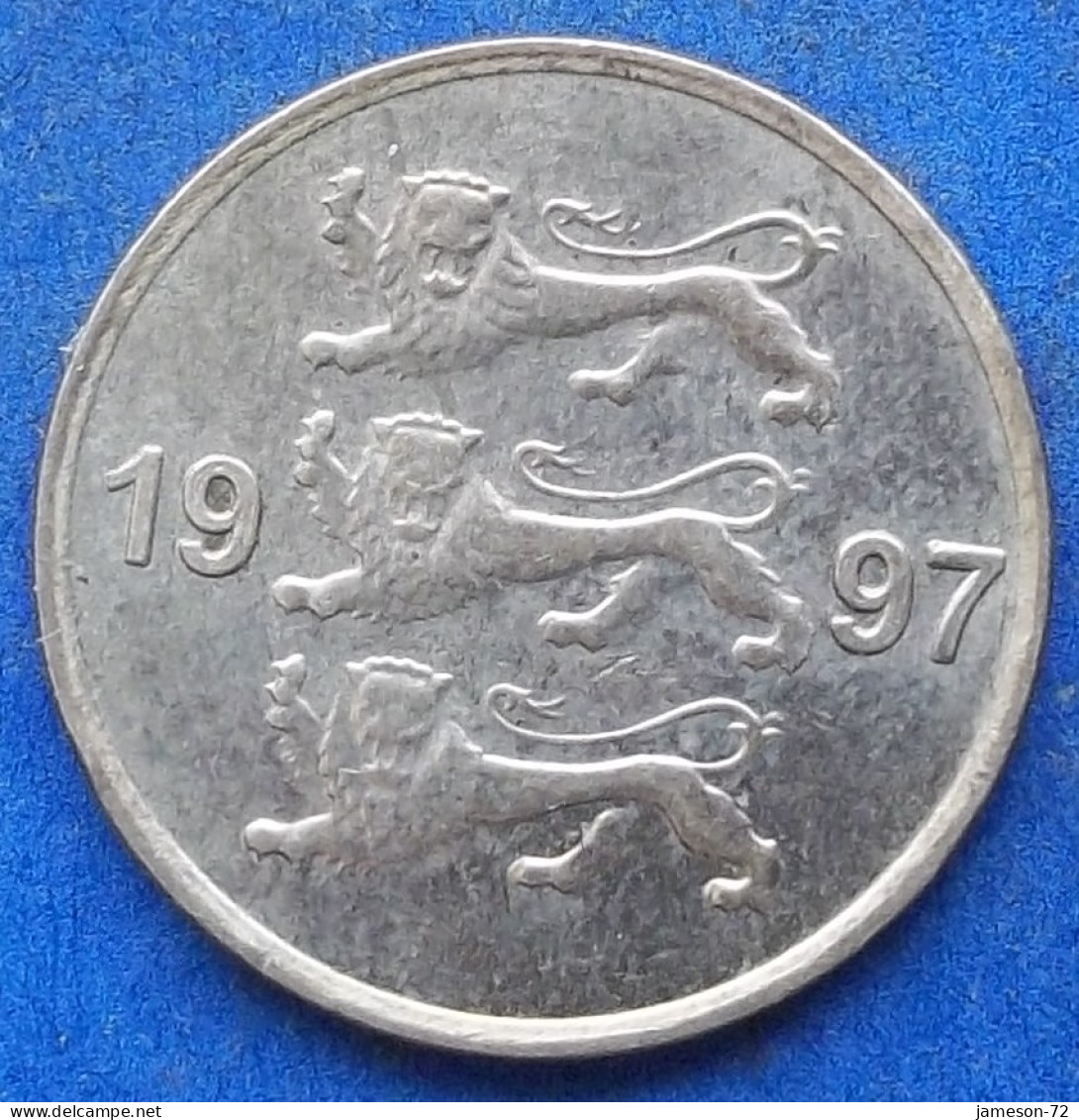This is a detailed close-up color photograph of a circular silver coin placed against a blue background. The coin, which occupies the entire image, features three medieval lions in a three-quarter view, their heads turned to the left. Each lion has a full mane, raised paws, and long, semi-curled tails that arch back over their bodies. The lions appear to be walking and growling, with their mouths open. The coin shows the numbers "19" on the left and "97" on the right, suggesting the year 1997. It has a pronounced ridge around the edge and a flat, beveled border. The image background includes text on the bottom left that reads "www.delcamp.net" and on the right "Jameson 7-2." Overall, the coin appears to be in relatively good condition and uncirculated.